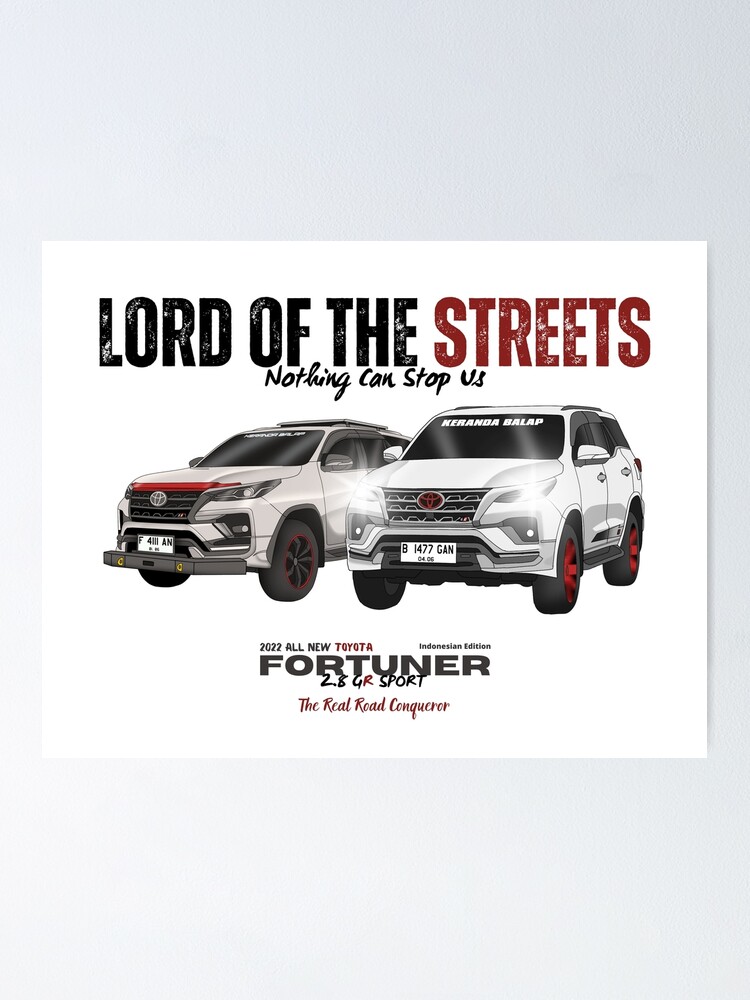The image depicts an advertisement set against a gray background with a scanned picture in the middle. The advertisement prominently features the text, "Lord of the Streets" at the top, with "Lord of the" in black font and "streets" in red. Below, in black letters, it declares, "Nothing can stop us." 

The central image shows two Toyota SUVs styled in a 3D cartoon-like graphic, with red accents around the black wheels. Both vehicles have the Toyota emblem and appear to be models from the 2022 all-new line. The specific model is the Fortuner 2.8 GR Sport, indicated as the "real road conqueror" at the bottom. The ad also mentions that this edition is tailored for the Indonesian market. Although some writing is partially visible on the windshields, it is difficult to read. Overall, the design emphasizes the robustness and versatility of the SUVs, appealing to potential buyers looking for a capable and stylish vehicle.